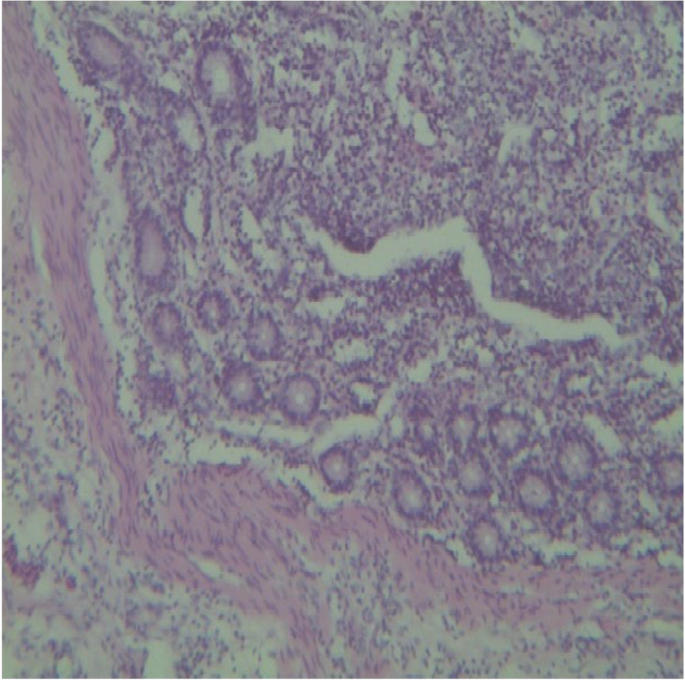The image appears to be a square, grainy, possibly digital creation or an abstract terrain-like representation that might evoke the imagery of a microscope slide. Dominated by different shades of creamy green and dark pink or purple, the composition includes many small dots, circles, and lines. Prominently featured is a swooping pink area flowing diagonally from the top left to the bottom right. This swoop is bordered by darker purple lines and dotted with purple granules. The lower left corner and areas surrounding the swoop display a creamish haze and collections of dense purple dots. The top right corner features a textured mesh of purple and white granules, adding to the overall vague and possibly cellular appearance. The collective lack of identifiable features such as text or figures makes the true nature of the image ambiguous, inviting interpretations from satellite imagery to cellular structures.